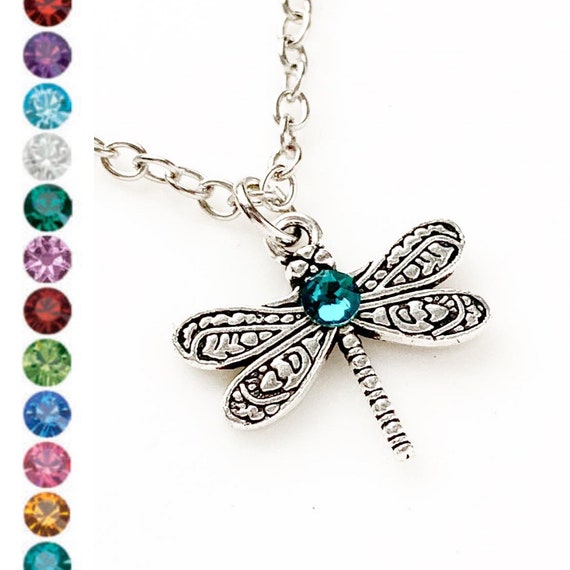The image displays a silver necklace centered on a pure white background, emphasizing its details. The necklace features a finely crafted dragonfly pendant with black-accented wings and body. The dragonfly has an aquamarine gem set in its center, adding a touch of vibrant blue. The chain is composed of linked silver rings, with the pendant hanging from a larger ring connected to the chain. To the left of the necklace, there's a radiant arrangement of circular gems, likely representing birthstones, that appear to burst outward. These gems vary in color, including shades of red, purple, teal, white, green, blue, pink, orange, and more. The overall perspective of the image is taller than it is wide, suggesting the careful layout of the jewelry and gems on a likely cropped or carefully staged background.